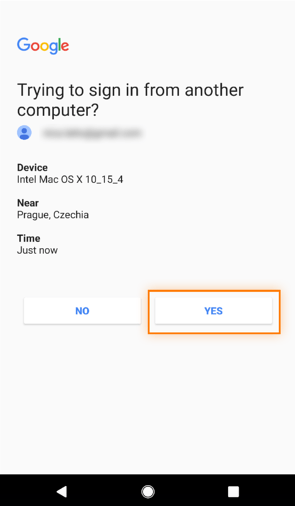The image depicts a partially cropped screenshot of a notification on a smartphone. At the top left corner, there's a Google icon, followed by a message that reads, "Try to sign in from another computer?" Next to this, a generic blue profile icon is visible, with the associated name completely blurred out. Below the message, detailed device information is provided: "Device: Intel, Mac OS X 10_15_4" and the location "Near Prague, Czechia." The timestamp is marked as "Just now."

Beneath the device details, there are two response options: "No" and "Yes." The "Yes" button is notably highlighted with a thin bright orange rectangle, indicating it has been marked for emphasis by someone. Further down, the image captures the phone's navigation bar—a simple black bar featuring a back triangle, a white circle, and a white square in the middle.

Conspicuously absent are typical notification icons such as the battery meter and time, suggesting that the screenshot might be incomplete or intentionally cropped. This image could originate from an instructive site or be edited using a photo application, but the exact context remains unclear.